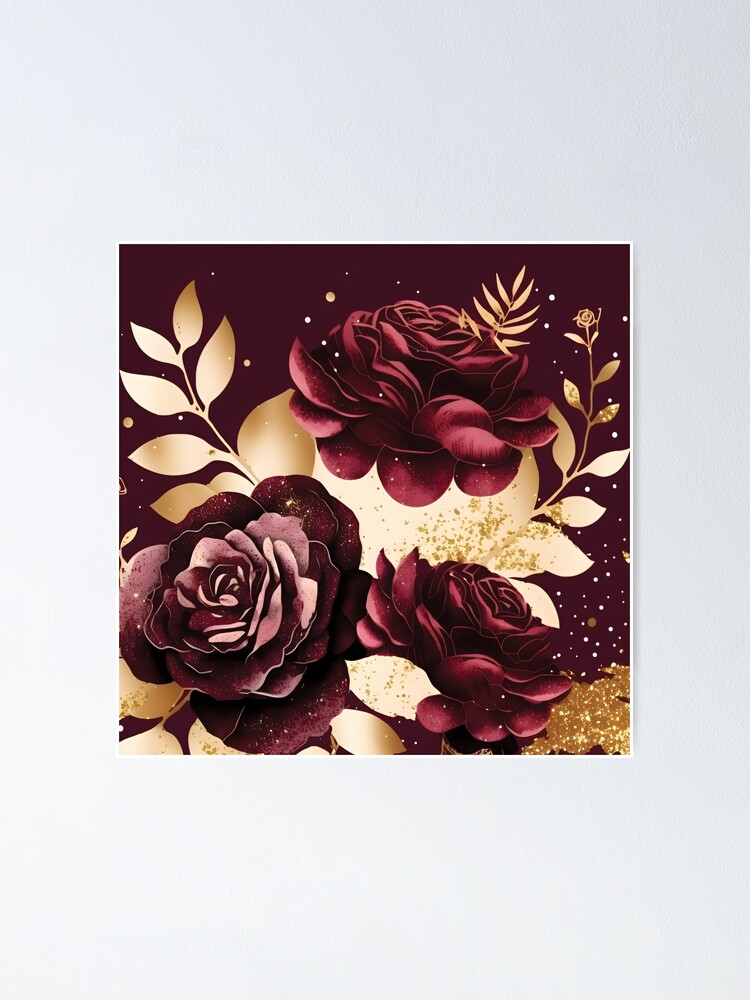This image appears to be a highly detailed photorealistic painting or digital art of three dark red roses without stems. The flowers are carefully arranged with one facing the camera at the bottom left, another at the bottom right, and a third positioned near the top, facing diagonally up and to the right. Behind the roses, there are ethereal leaf shapes with a gradation of gold and white hues, lending a decorative and somewhat ethereal appearance. The background is a rich, deep maroon that borders and highlights the entire composition. Additionally, white speckles are scattered throughout the image, most prominently on the right side and top left, adding a layer of texture and intricacy. A notable gold glittery patch is located at the bottom right, adding a touch of sparkle to the overall artwork.